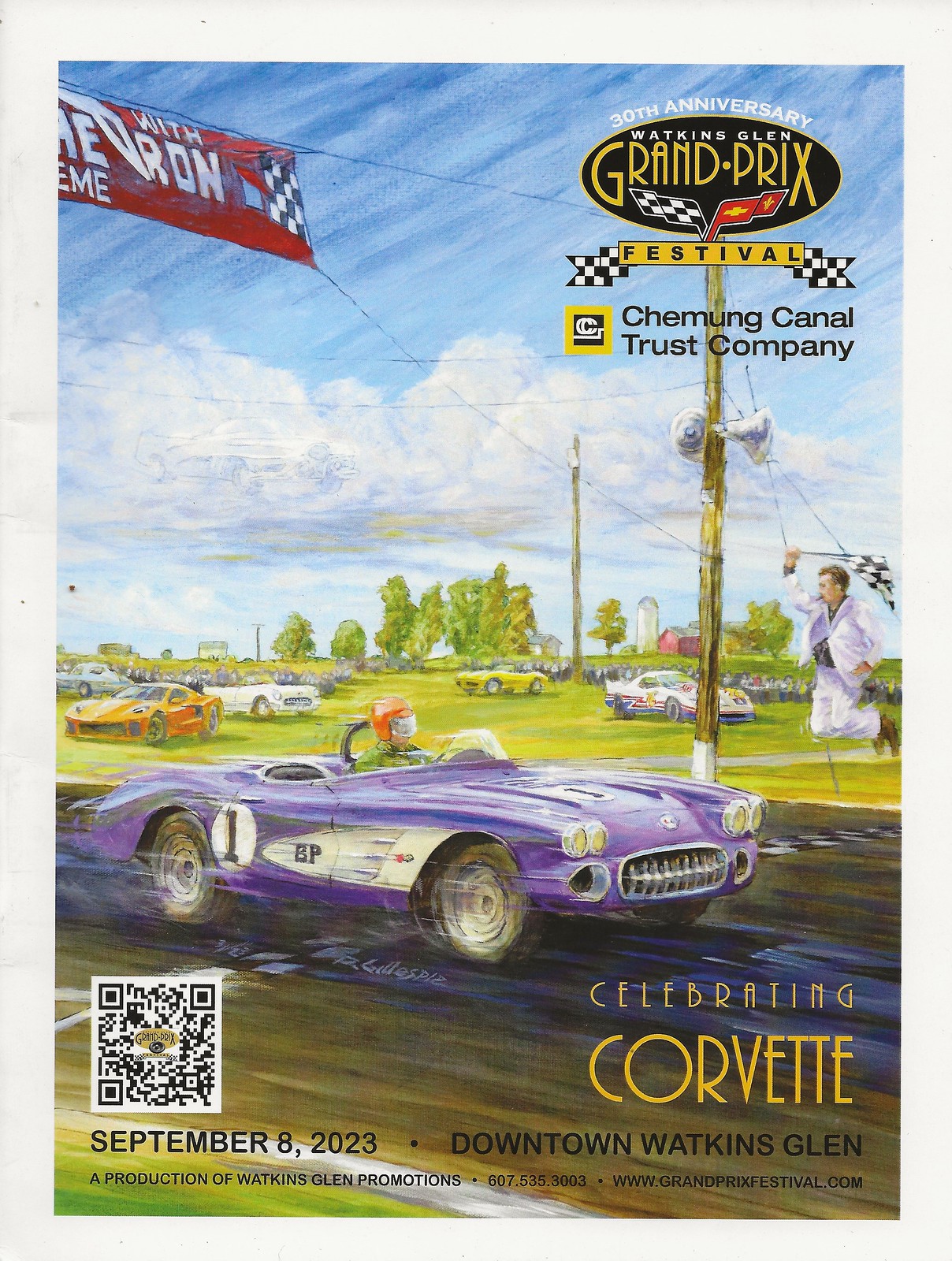This detailed cover illustration for the 30th Anniversary of the Watkins Glen Grand Prix Festival, sponsored by Chemung Canal Trust Company, depicts a dynamic racing scene. Dominating the foreground is a purple Corvette race car, labeled with the number one, speeding past a checkered finish line. The car's driver, distinguished by an orange helmet, is captured mid-race as a man in a white suit and purple shirt energetically jumps in the air to wave the checkered flag, signifying victory. Surrounding the track, multiple cars are visible against a backdrop of grassy fields, trees, and a vivid blue sky dotted with white clouds.

In the upper right corner, a prominent black and yellow sign announces the festival's 30th anniversary, with “Watkins Glen” in bold white letters above “Grand Prix” accompanied by racing flags and a banner stating "Festival." Below this, the sponsor's name, Chemung Canal Trust Company, is displayed. 

At the bottom left, further details include a QR code, the date "September 8th, 2023," and the note "Celebrating Corvette." Additionally, the text "Downtown Watkins Glen" and "A production of Watkins Glen Promotions" alongside a phone number and website provides additional event information.